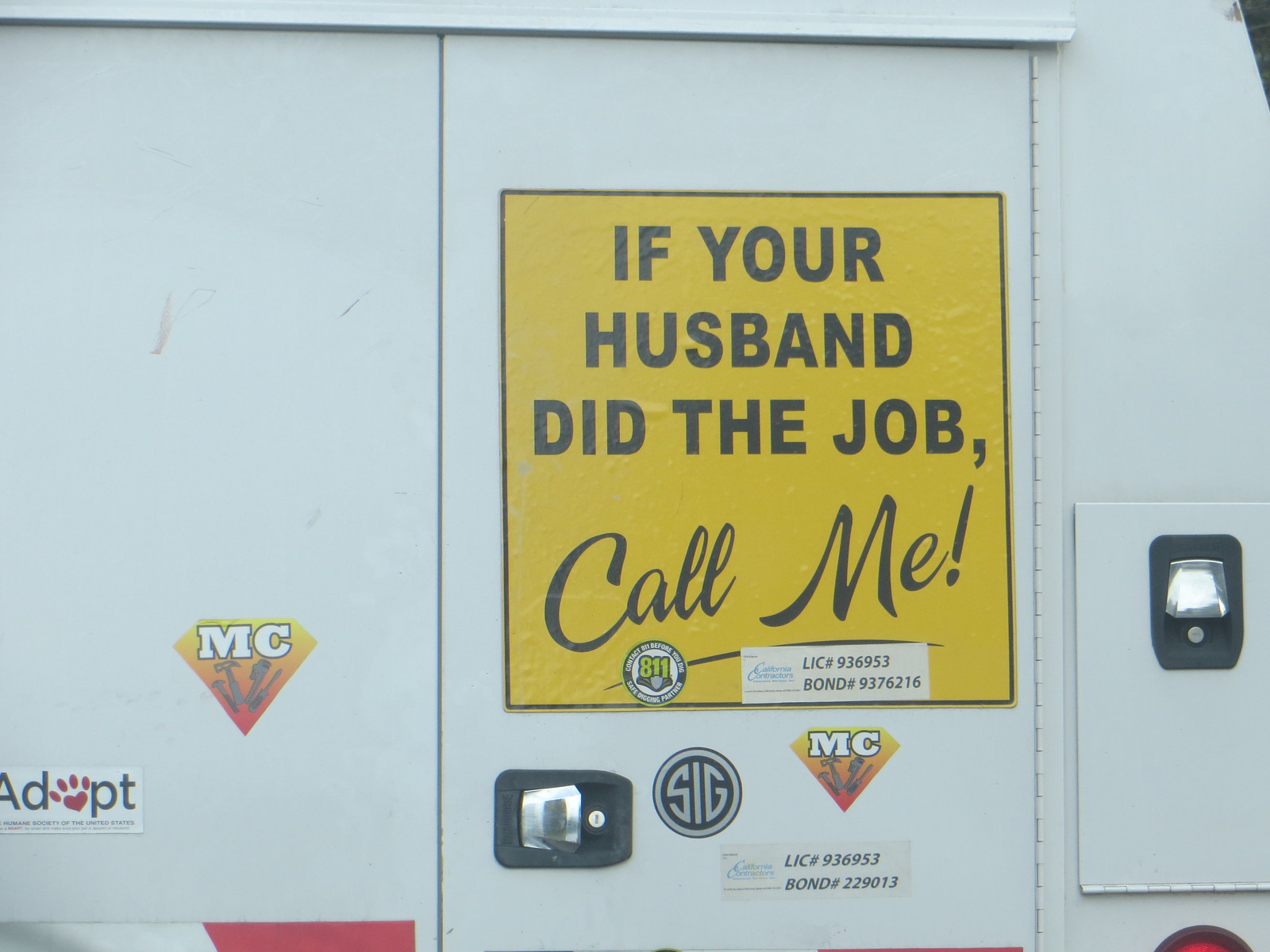The image features a door on a white background. Prominently displayed in the center is a yellow sign with black lettering that reads, "If your husband did the job, call me." Beneath this message, there are numbers, including a license number "936953" and a bond number "9376216." Directly below the main text, there is a diamond-shaped sticker with tools depicted and large white letters that say "MC." To the left side, there's another circle-shaped sign that has "SIG" in gray lettering with a black border. Further to the left, there is black text saying "adopt" with a pet paw replacing the letter "O". On the right side of the door, there is a small, silver, hooded container mounted on the wall that resembles a sanitizer dispenser or a dropbox.